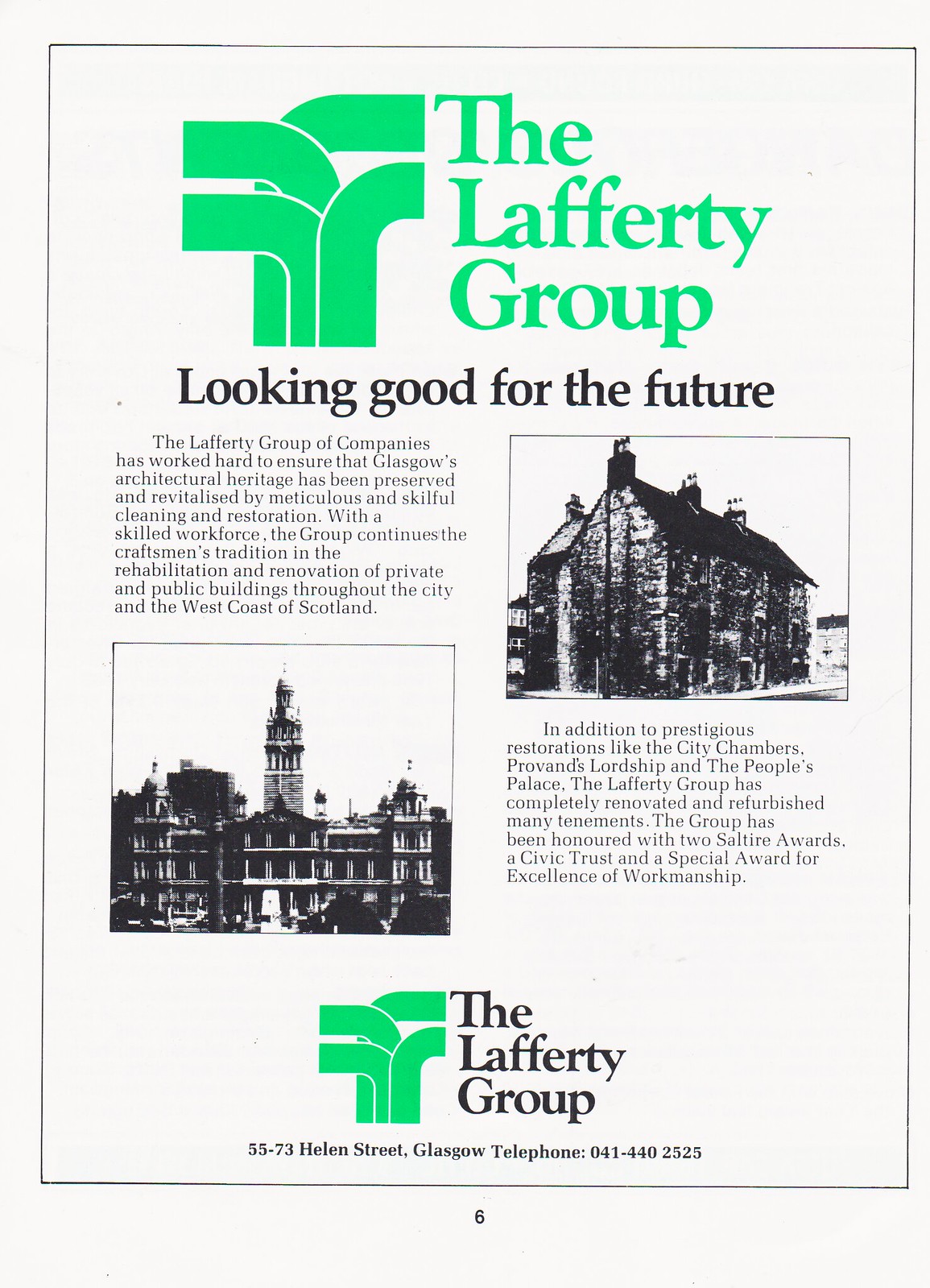This appears to be a scanned advertisement page from a magazine or printed program for the Lafferty Group. The page is slightly off-white, featuring images, text, and logos primarily in black, with some elements in green. At the top, there is a prominent green interlocking, curved logo beside the name "Lafferty Group" in bold green text. Below, a tagline in black reads: "Looking good for the future."

The advertisement includes two black-and-white images of buildings, diagonally positioned with one in the upper right corner and another in the lower left. The upper right image depicts a very old, large stone building with multiple chimneys, while the lower left image shows a slightly more modern building featuring large towers in its center and corners.

The accompanying text describes the Lafferty Group's commitment to preserving and revitalizing Glasgow's architectural heritage through meticulous and skillful cleaning and restoration by a skilled workforce. It highlights notable projects such as the restorations of the City Chambers, Provence Lordship, and the People's Palace. The group is celebrated for its craftsmanship in renovating private and public buildings throughout Glasgow and the west coast of Scotland, having received prestigious awards including two Saltire Awards, a Civic Trust Award, and a Special Award for Excellence in Workmanship.

At the bottom center of the page, the Lafferty Group logo reappears, this time in black, with accompanying text: "55-73 Helen Street, Glasgow. Telephone 041-440-2525." The very bottom of the page shows the number 6, likely indicating a page number.